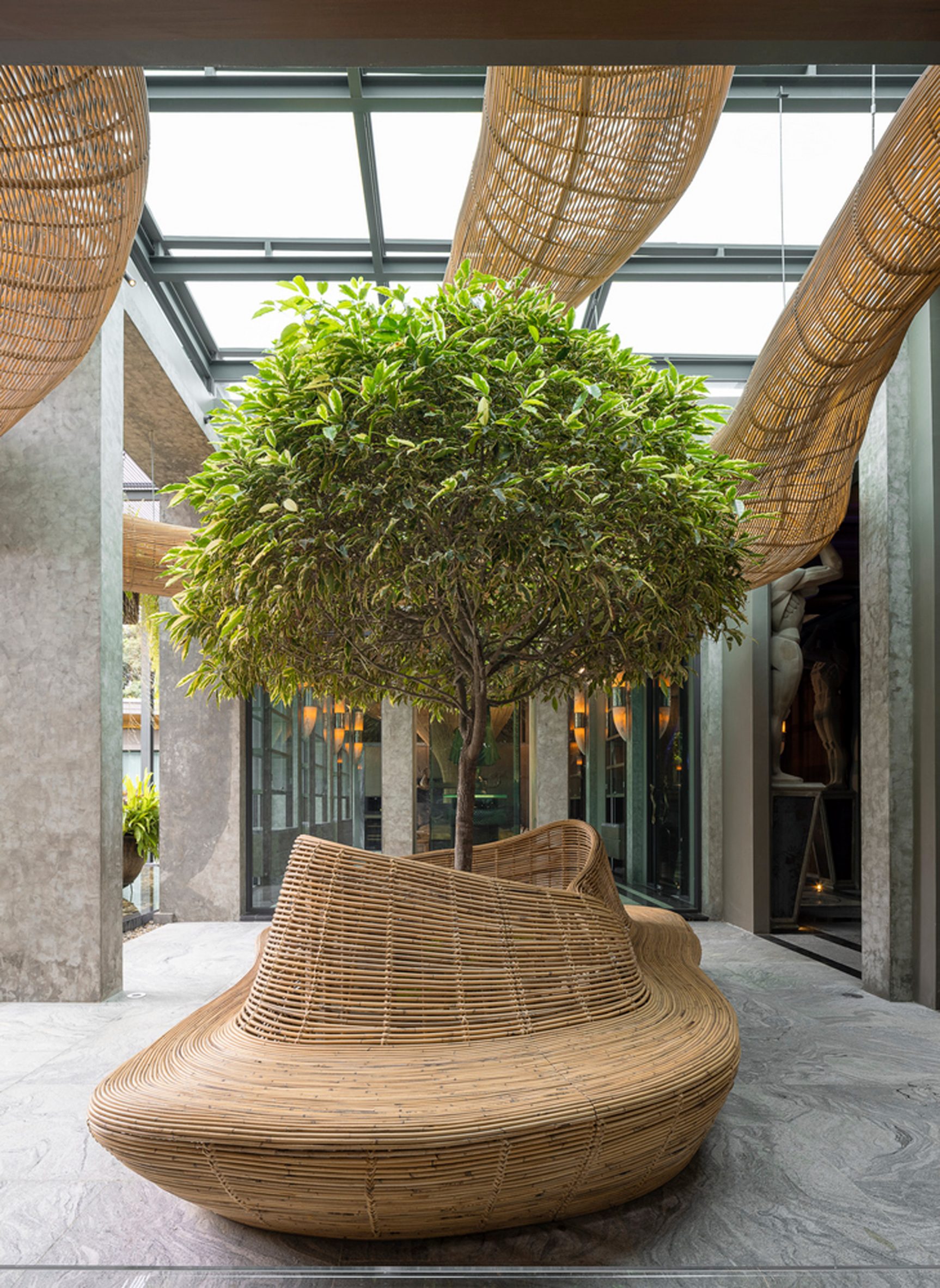The image captures a modern, minimalist architectural exhibit filled with natural and contemporary elements. Dominating the scene is a striking, large wooden vase-like structure with a wicker basket texture, shaped somewhat like an elongated boat with an open top. Emerging from its center is a thin, young tree with green leaves and brown bark. The setting appears to be inside a museum or architectural design exhibit, evident from the open steel-framed roof with numerous windows that allow natural light to flood the space. Surrounding the main structure, additional wicker basket forms hang from the ceiling, and the floor is a light gray concrete slab. In the background, there's a composition of windows and doors adorned with gray and yellow striped lights, enhancing the modern ambiance. The space includes various sculptural elements and stone pillars, lending a touch of sophistication and artistry to the overall design.